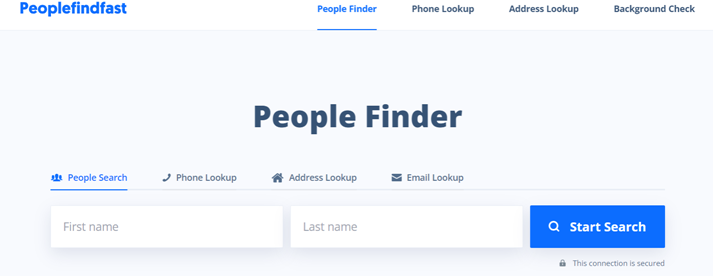The left side of the image showcases the text "People Finder" in blue lettering. To the right, a vertically stacked list includes "People Finder," "Phone Lookup," "Address Lookup," and "Background Check" with "People Finder" highlighted in blue. Below this list, there's a light blue rectangle containing "People Finder" written in bold black lettering. 

Beneath the rectangle, "People Search" is displayed along with an icon depicting three people's heads in blue. Adjacent to it on the right, "Phone Lookup" is written next to an icon of a phone. Further right, "Address Lookup" is accompanied by an icon of a house, and "Email Lookup" is next to a piece of mail icon, all in black lettering.

Below these icons, there are two white input boxes. The first one is labeled "First Name" in gray lettering, and the second one is labeled "Last Name," also in gray. To the right of these input boxes, a blue button with the text "Start Search" in white lettering is displayed, featuring a white magnifying glass icon to the left of the text. Below this section, there’s an image of a lock with the text "This connection is secured." Central on the page, "People Finder" appears prominently in bold lettering.